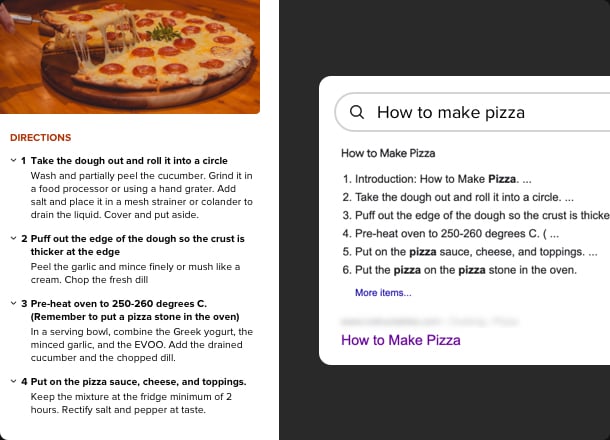The image showcases a detailed webpage on how to make pizza. At the top, there is a search input field with the query "how to make pizza." Immediately below the search bar, the text "How to make pizza" is slightly bolded, emphasizing the topic. The next section introduces the instructions, starting with a subtitle "Introduction, How to make pizza" where the word "pizza" is in bold. 

Following the introduction are numbered steps for making pizza:
1. Take the dough out and roll it into a circle.
2. Buff up the edge of the dough so the crust is very thick.
3. Preheat the oven to 250-260 degrees Celsius.
4. Put on the pizza sauce, cheese, and toppings.
5. Place the pizza on the pizza stand in the oven.

Additionally, there is a hyperlinked text in blue labeled "more items," and below this, the phrase "how to make pizza" appears again in purple.

On the left side of the webpage, there are more detailed instructions with a corresponding image of a pizza at the top. Directions are highlighted in red text and include the following steps:
1. Take the dough out and roll it into a circle, followed by additional instructions.
2. Puff out the edge of the dough to create a thick crust, with further instructions beneath.
3. Preheat the oven to 250-260 degrees Celsius before placing the pizza in the oven, with more guidance included.
4. Apply the pizza sauce, cheese, and toppings, followed by further steps to complete the process.